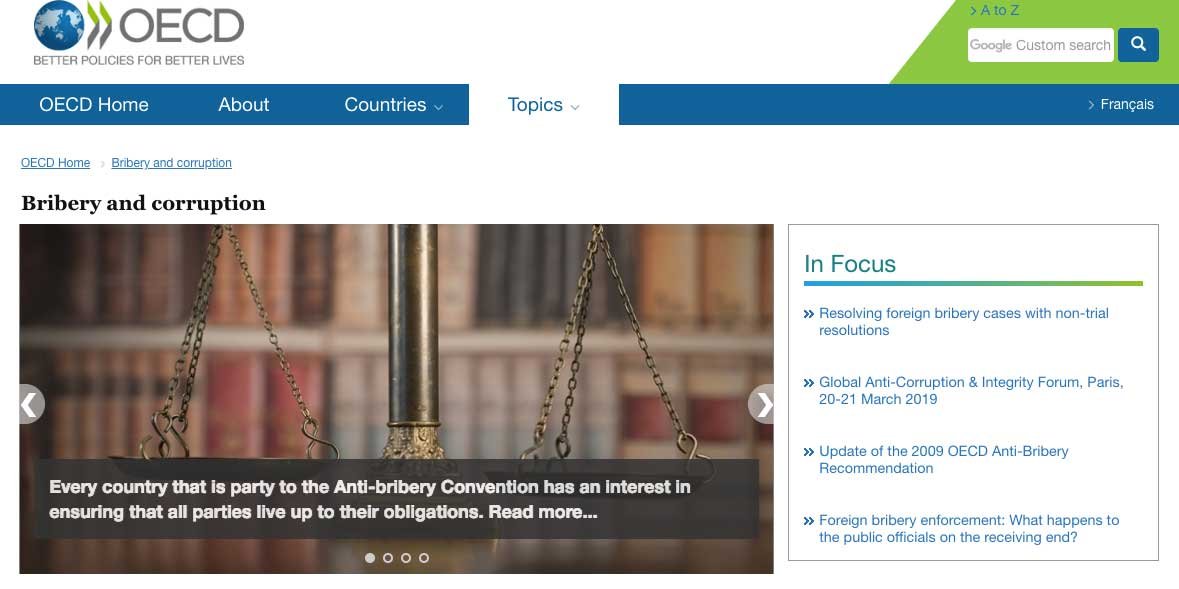This is a cropped screenshot of an OECD (Organisation for Economic Co-operation and Development) webpage. At the top left corner is the recognizable OECD logo. To the right, a green box, distinguishably slanted on its left side, displays "A to Z" at the top, accompanied by a drop-down menu. Below this, a search bar prominently labeled "Google Custom Search" in small grey letters, is situated, with a blue magnifying glass icon immediately to its right for initiating searches.

Beneath this search section, a blue navigation banner spans across the screen, offering various options. The menu starts with "OECD Home" followed by "About" and "Countries," each with a drop-down box. "Topics," also paired with a drop-down option, is currently selected, setting the visible content area to the "Topics" tab. The main content area boasts a clean, white background.

On the left side of the page, there is an image with the title "Bribery and Corruption" above it. The bottom of the image is overlaid with a black bar containing a descriptive caption. Flanking the image, small grey arrows on either side facilitate scrolling through additional photos.

To the right of the image, there’s a box titled "In Focus." Within this section, clickable article titles are neatly listed, providing quick access to key articles on the topic.